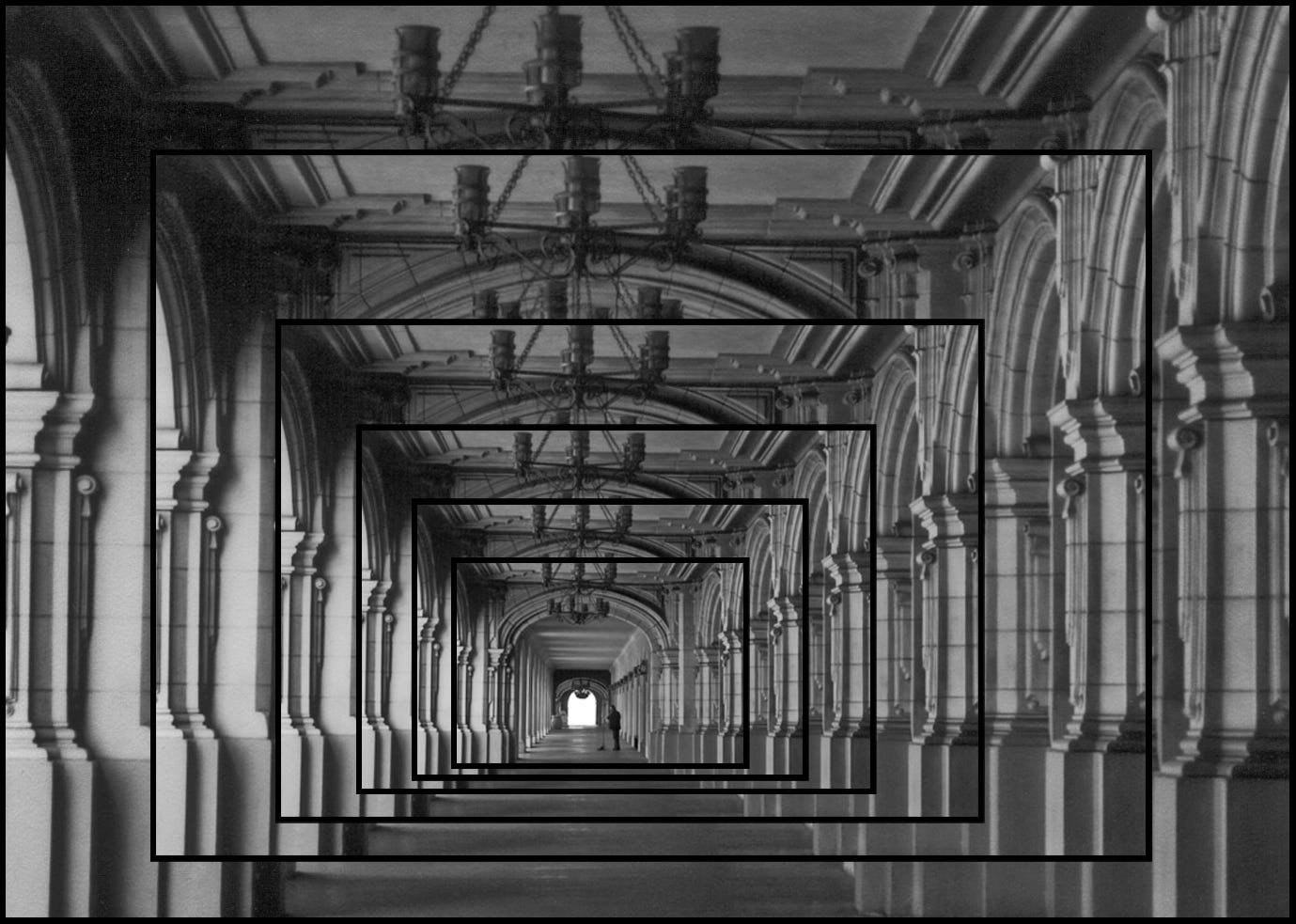This black-and-white image captures the ornate interior of a long corridor within a historical building, possibly from the early 1900s. The corridor is lined with concentric columns on both sides, featuring intricate stone archways that create a patterned, almost mirrored effect, which enhances the sense of depth. High above, multiple chandeliers dangle, their lights casting a faint glow that accentuates the architectural details. The repeating rectangular forms and the symmetry of the columns suggest a repeated or patterned photograph, adding an artistic layer to the depiction. The corridor stretches far into the distance, culminating in what appears to be a large open window, giving a glimpse of the outside. In the distance, a solitary figure can be seen sweeping the floor, contributing to the tranquil and timeless atmosphere of the scene.